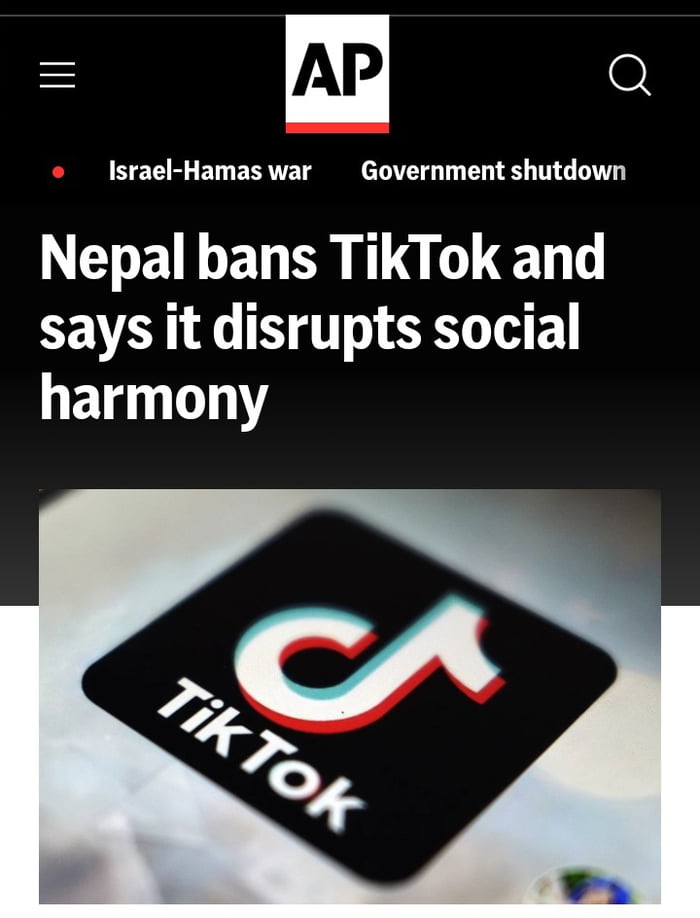A sleek website splash page for an article by the Associated Press (AP) features a predominantly black background. Centered at the top is a black box displaying the iconic AP logo: the letters "A" and "P" in black, set against a white square with a red underscore at the bottom. To the right of this logo is a search function, and to the left is a hamburger menu. Directly beneath these elements are clickable indicators for various news topics, with "Israel-Hamas war" and "government shutdown" being two of the options presented.

Below the navigation, the headline for the featured article reads, "Nepal bans TikTok and says it disrupts social harmony," in bold white text set against the black background. The visual centerpiece of this section is an image overlapping both the black and an adjoining white background. This image showcases the TikTok logo, as seen on a mobile app screen, featuring the iconic musical note symbol and the word "TikTok" in white with a shallow depth of field, adding a touch of sophistication and focus to the presentation.